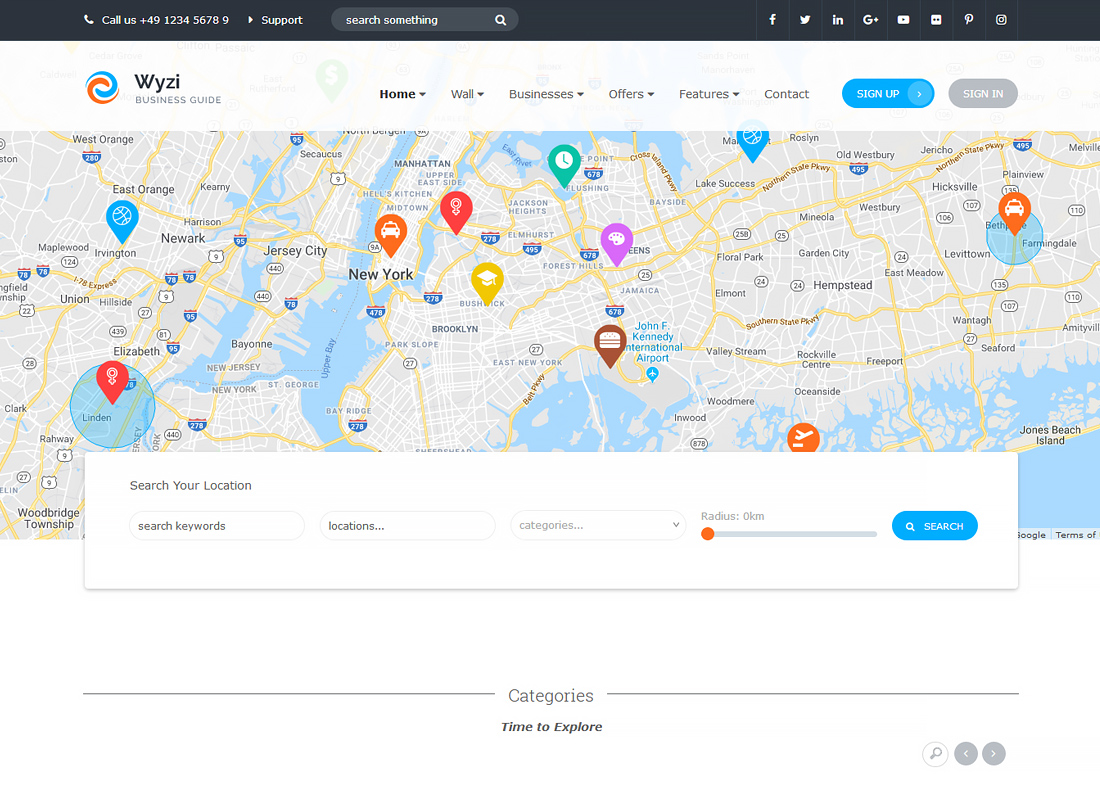In this image, we see a detailed website interface overlaying a map of various locations. The top left corner features a "Call Us" prompt with the phone number +49 123 456 789, accompanied by options for support and a search bar where users can type queries. In the top right corner, the website provides a series of social media links, including icons for Facebook, Twitter, LinkedIn, Google Plus, YouTube, Pinterest, Instagram, and Discord.

The map itself highlights several key locations such as Manhattan, Upper East Side, Hell's Kitchen, New York, Jersey City, St. George, Upper Bay, Shreveport, Hempstead, East Middle, Garden City, and Floral Park. Additionally, various pins mark specific areas, color-coded in shades of blue, purple, brown, red, orange, gray, and white, indicating different points of interest or significance on the map.